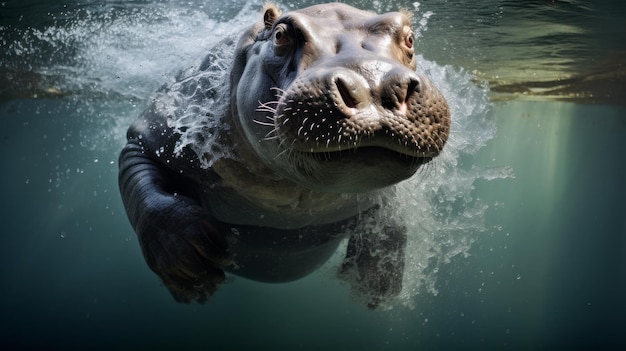The image depicts a dark gray hippopotamus swimming underwater. Its prominent nostrils and brown eyes are visible through the water. The hippo resides in a dual-toned aquatic environment, where the water is a dark blue-green shade, transitioning to a greener hue towards the surface. White water splashes against the side of its body, accompanied by clear and white bubbles. Light filters through the surface on the right side, casting a gentle illumination across the scene. Additionally, the hippo's whiskers are white, and it has brown ears and brown patches around its eyes. The chest appears lighter in color, either white or a lighter gray, contrasting the darker gray of the rest of its body. The overall aesthetics suggest a painterly or digitally created image rather than a photograph.